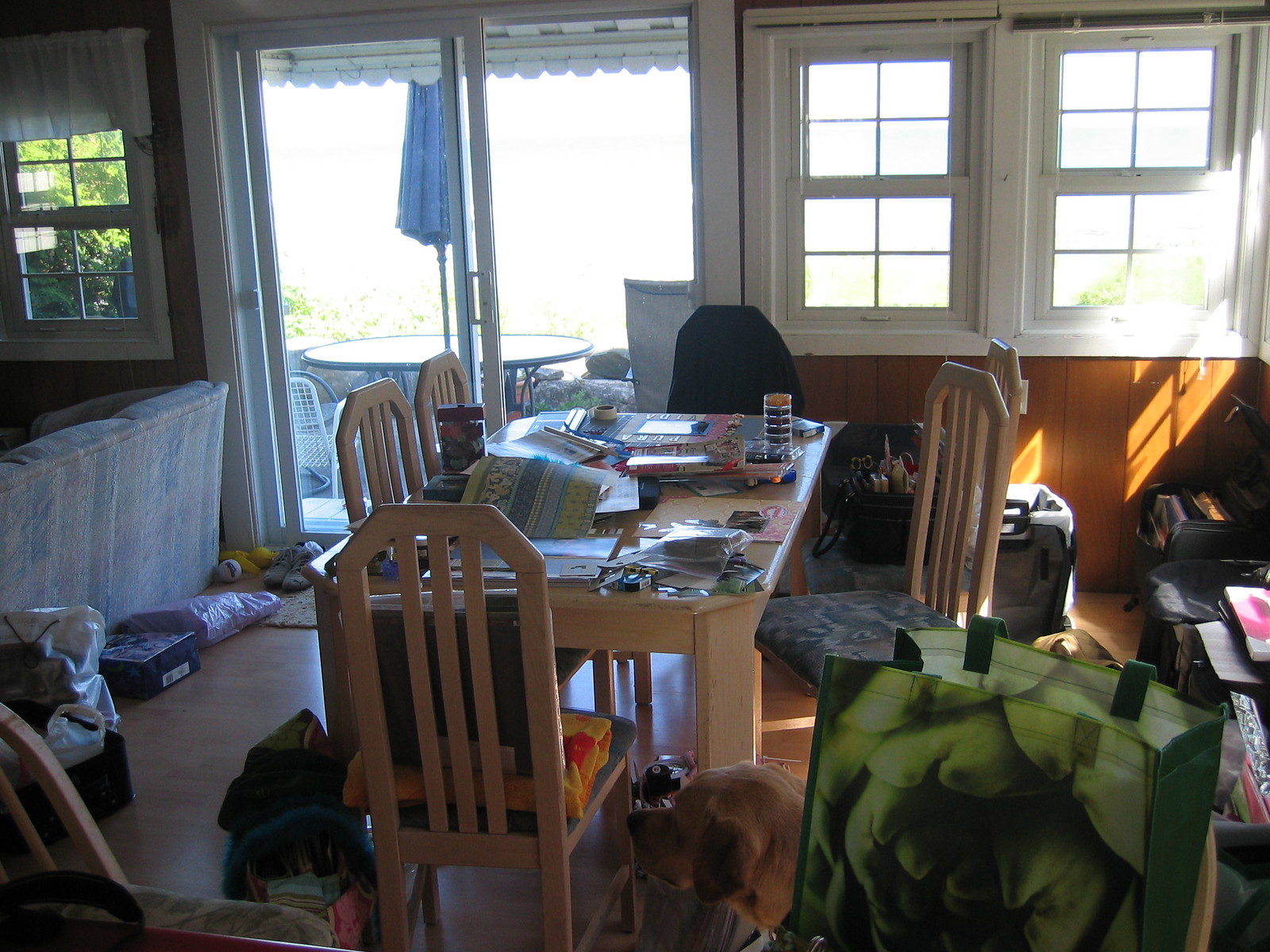In this photograph of a dining room, you can observe a room teeming with activity and clutter. Central to the image is a blonde wooden dining table, cluttered with an array of items including papers, maps, canisters, drinking glasses, and placemats. Surrounding this table are four matching blonde wooden chairs, alongside an additional office chair positioned at the table's end. A patterned cushion adorns one of the chairs on the near side.

On the room's far side, an abundance of natural light pours into the room through two large, brightly illuminated windows, flanked by a sliding glass door that opens to the outside. Visible through these glass doors is an outdoor table encircled by chairs, a hint of greenery, and a blue umbrella providing a pop of color.

The floor around the dining area is scattered with miscellaneous items such as bags and boxes, adding to the room's busy atmosphere. A brown dog can be seen lounging amidst this clutter. To the left, the room transitions into what appears to be a living room, with the edge of a multicolored dark couch and another window that offers a view of the greenery outside. The photograph captures the lived-in, dynamic nature of this home space, where daily life and activity are in full swing.